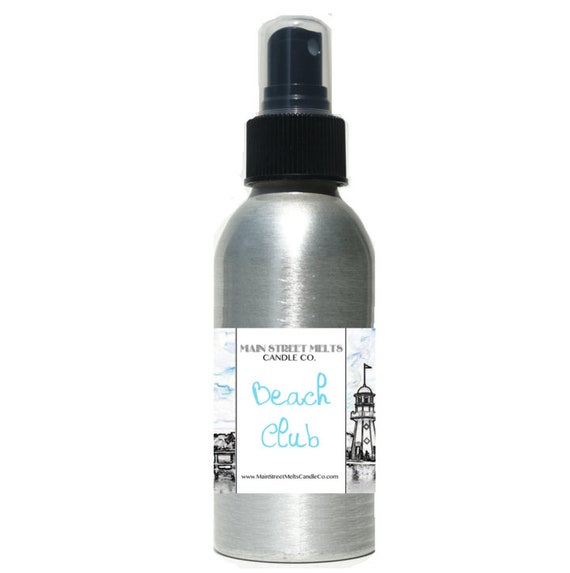The image is a detailed close-up photograph of a silver spray bottle, likely made of brushed aluminum or steel, designed for candles. This bottle features a black spray nozzle covered by a clear plastic cap. The front label is primarily white and prominently displays the brand "Main Street Melts Candle Co." in silver and black text, with the product name "Beach Club" written in cursive blue lettering within a white rectangle that appears hand-drawn. Beneath this, the URL "www.mainstreetcandleco.com" is printed in black. The label also includes illustrations: on the left, a cliff edge, and on the right, a lighthouse with a flag on top, rendered in black, white, and gray. Above these illustrations, a cyan sky with white accents wraps around the top of the bottle. The background of the image is plain white, emphasizing the bottle at its center.